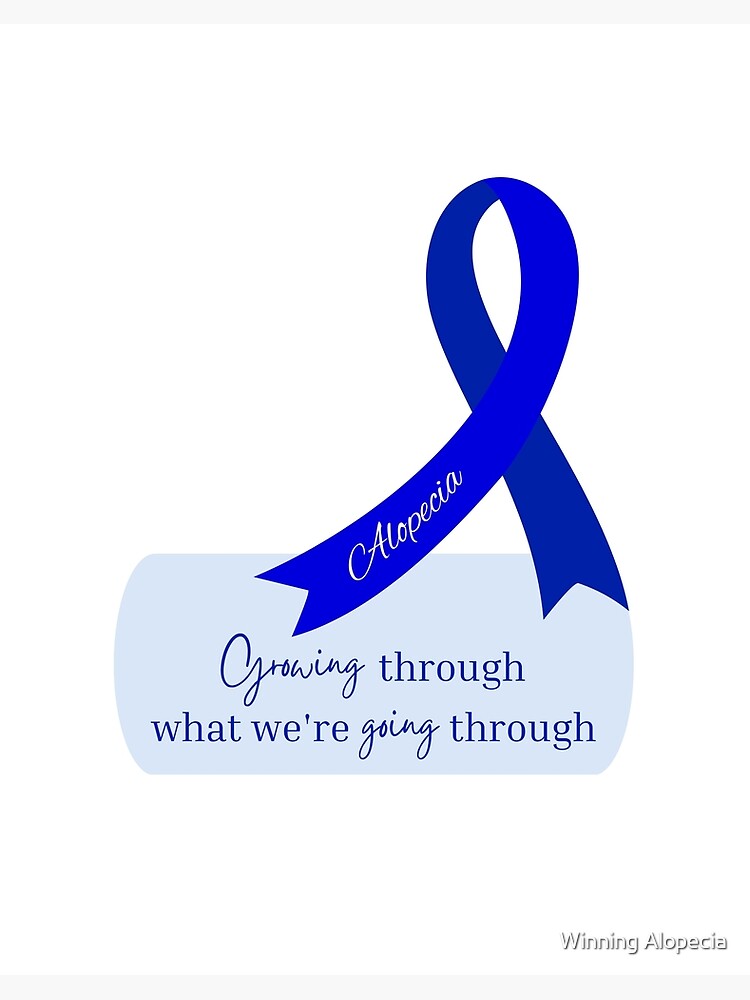The image features a prominent blue ribbon with the word "Alopecia" written in white text on the left side, symbolizing support for those experiencing hair loss. Below the ribbon is a rounded blue rectangle containing the inspirational phrase, "Growing through what we are going through," with the words "growing" and "going" elegantly styled in a handwritten script, while the rest of the phrase is in a simple, lowercase font. This design rests on a clean, white background and is likely part of a logo or slogan for an Alopecia-related foundation or charity. At the bottom right corner, set against a very pale gray bar, the phrase "winning alopecia" is discreetly written in thin, faint black lettering, further emphasizing the message of resilience and support.